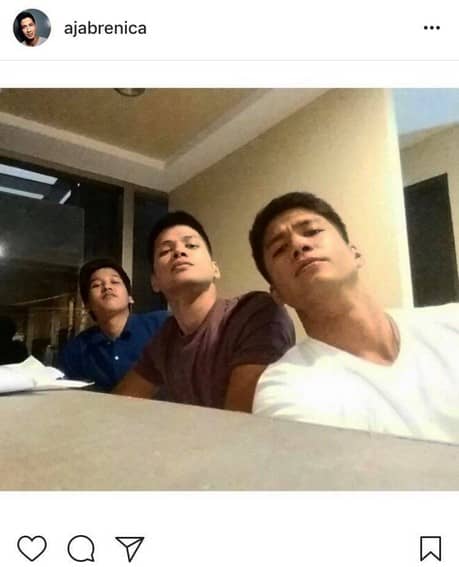In this Instagram post by AJABRENIC, the profile picture and account name are displayed in the top left corner. The main image features three Hispanic men seated at a gray desk, seemingly taking a selfie. All three are looking at the camera with neutral expressions. The man on the left wears a blue button-up shirt, the one in the center sports a brown short-sleeve t-shirt, and the man on the right has on a white t-shirt. Behind them, a beige wall with white trim and a window indicating nighttime can be seen. Papers are scattered on the desk in front of them.